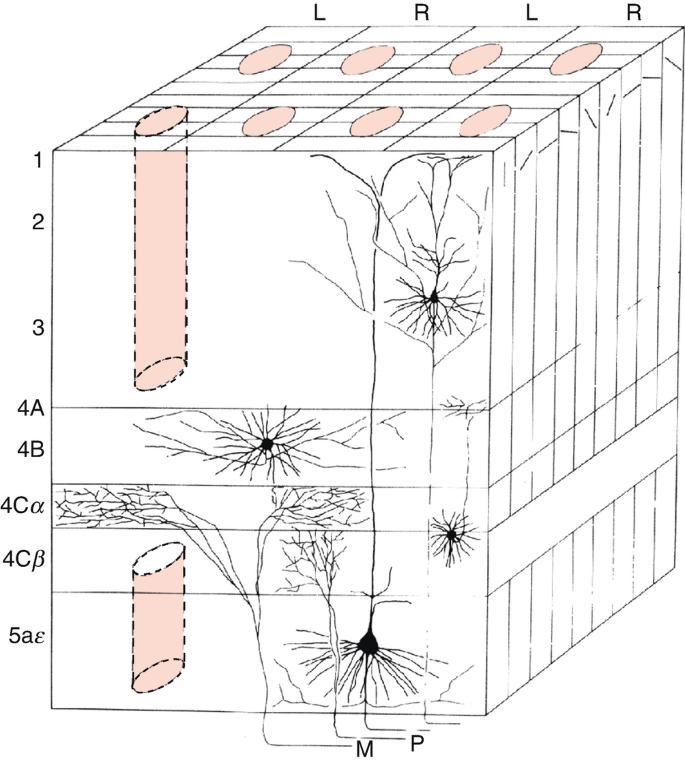This intricate black and white diagram features a cubical structure embellished with detailed line work and annotations. The cube has several vertical lines running down its right side and multiple horizontal lines on its front face, intersecting a large rectangular section. Soft pink shading highlights specific elements including two black-outlined cylindrical shapes on the left side—one more substantial at the upper left and a shorter one at the lower left.

The cube's interior is adorned with black geometric and organic shapes that resemble flowers with radial stems emanating from black centers, and some elements resemble spiders descending or ascending webs. The upper portion of the front face includes horizontal rows of pink ovals. The left face of the cube is systematically labeled with vertical numbering: 1, 2, 3, 4A, 4B, 4CA (alpha), 4CB (beta), and 5AE. 

Additional annotations are dispersed throughout, such as 'M' and 'P' on the front and 'L' and 'R' on the back side. These letters likely indicate specific parts or facets of the diagram. Overall, the image merges scientific precision with artistic complexity, presenting a multifaceted structure enriched with both geometric and organic elements.